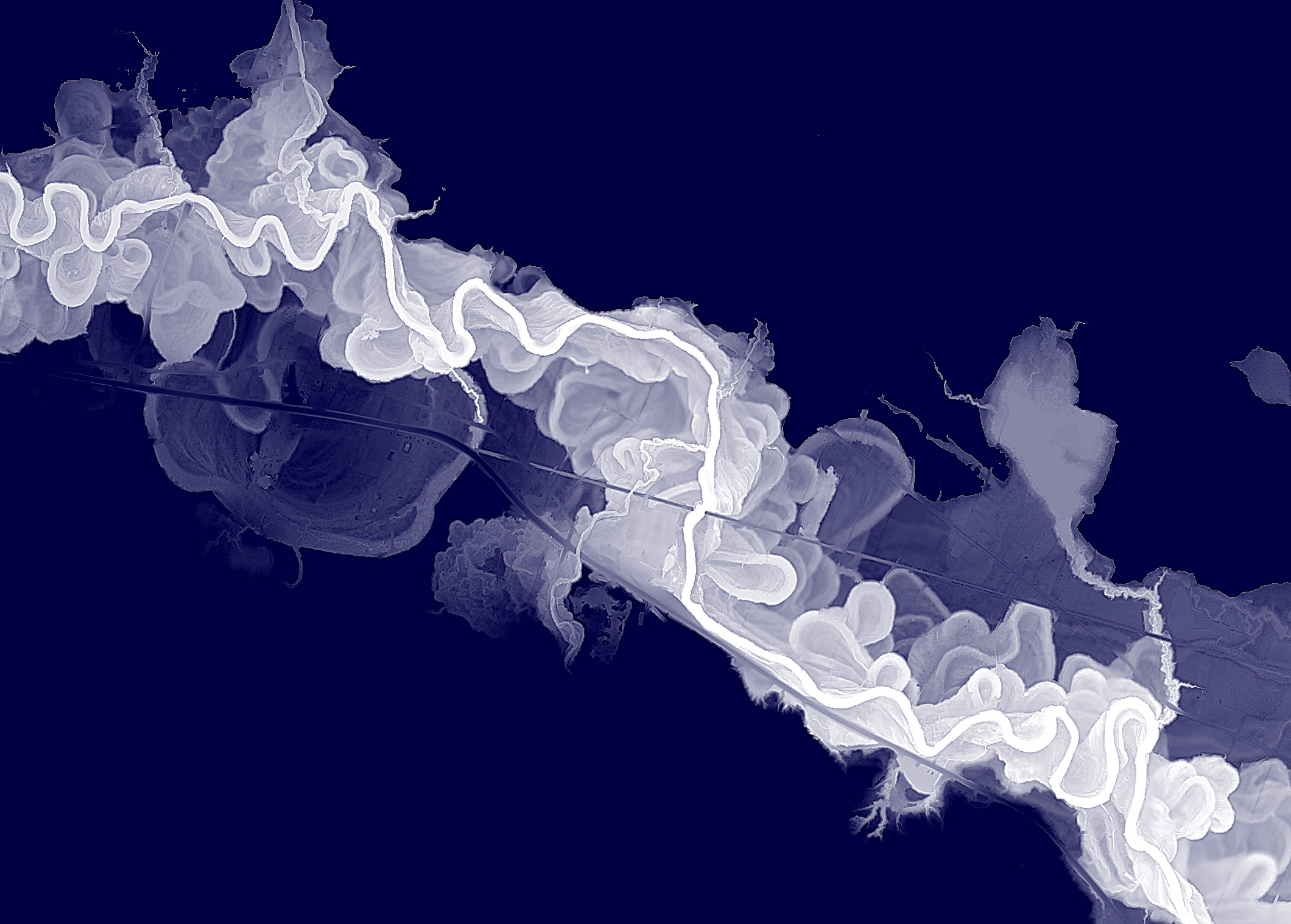The artwork is a captivating monochrome abstract image that features a dark blue background with a diagonal trail of swirling, silvery white smoke. The ethereal wisps and gaseous shapes meander from the top left corner down to the lower right corner, creating a fluid, spiraling motion. Throughout the image, the smoke varies in shades, with elements of translucent white, light bluish gray, and faint purples, adding depth and texture. The outer fringes of the smoke diffuse into the dark background, giving a sense of movement and softness. There are also darker streaks and horizontal lines interwoven into the design, suggesting a river-like flow. This intricate interplay of forms and hues creates a mesmerizing, immersive visual experience.